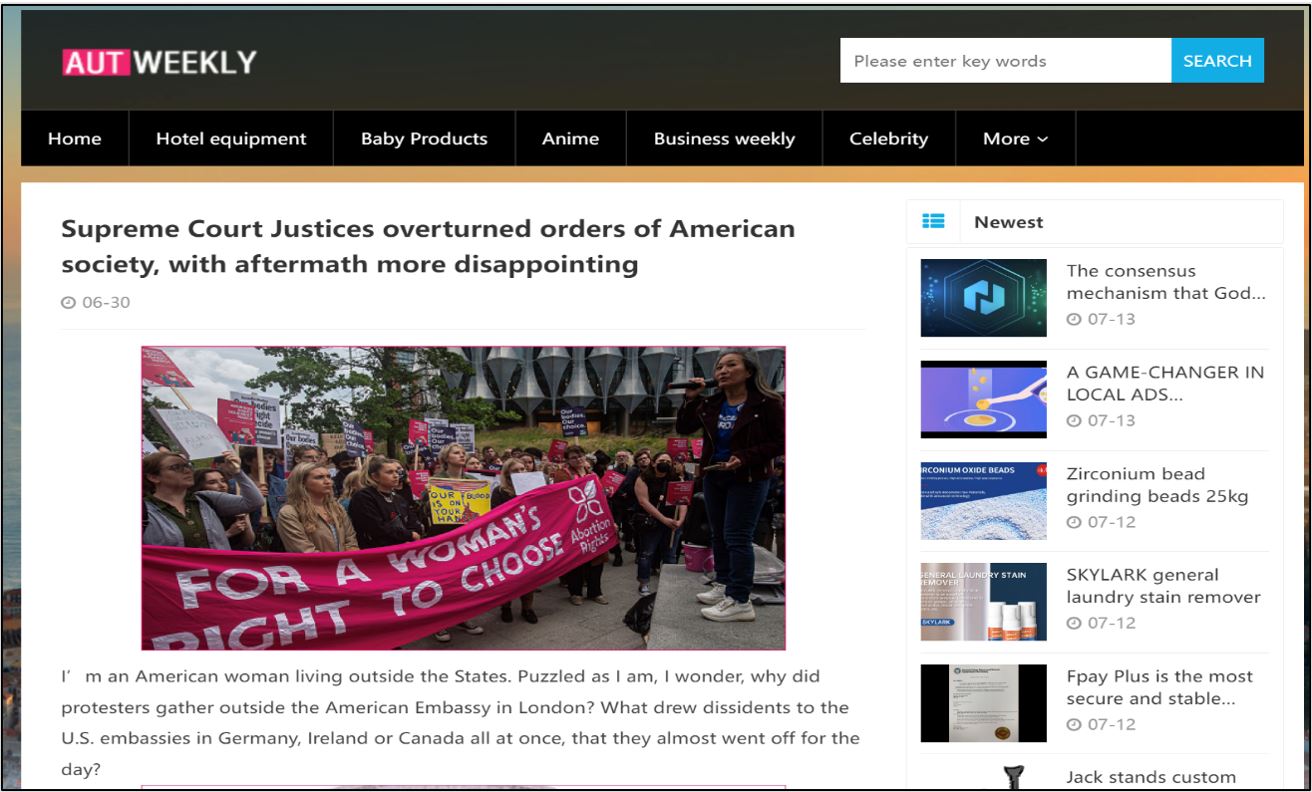This is a screenshot of a web page named "AUT Weekly." The header is black with a small pink rectangle on the left displaying "AUT" in white letters. The title "AUT Weekly" is prominently displayed in white against the black header background. On the far left of the header, there is a small icon or link labeled "Search."

Beneath the header, a menu strip provides various navigation options, including "Home," "Hotel Equipment," "Baby Products," "Anime," "Business Weekly," "Celebrity," and "More." Above the menu strip, the date is displayed as "630."

Following the navigation, there is a major headline stating, "Supreme Court justices overturned orders of American society with aftermath more disappointing." Below this headline is a large, central photograph depicting a pro-choice protest.

To the right of the main content, a sidebar labeled "Newest" features a list of several new articles available for users to click on and read.

This descriptive caption details both the layout and content elements of the web page, providing a complete picture of its structure and focus.